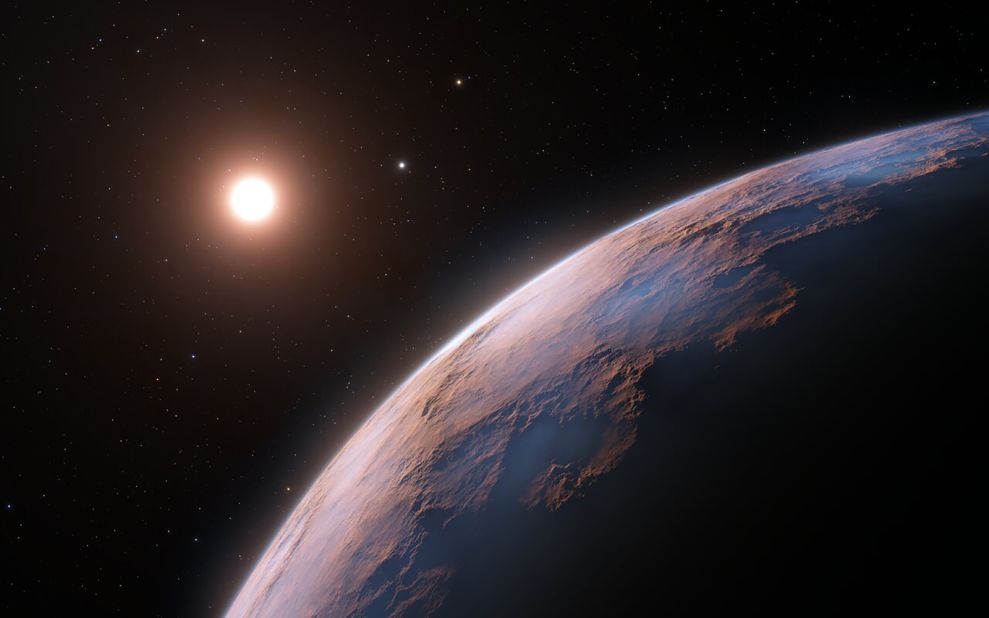This computer-animated image of outer space captures a vivid celestial scene. Dominating the lower right portion of the frame is a curved segment of a planet, identified as Earth, showcasing distinct brown landmasses and blue oceans without any traces of green. Above this terrestrial expanse, positioned towards the upper right, a luminous sphere believed to be the Sun casts a bright, somewhat hazy glow across the cosmic backdrop. Surrounding the planet and sun, the expanse of pitch-black space is dotted with several white specks, representing distant stars of varying sizes. Notably, a moon is included in the scene, appearing unusually close to Earth, though it is understood that this proximity is an artistic representation. The entire composition lacks any textual or numerical annotations, focusing solely on the celestial bodies and the dark, vast universe.